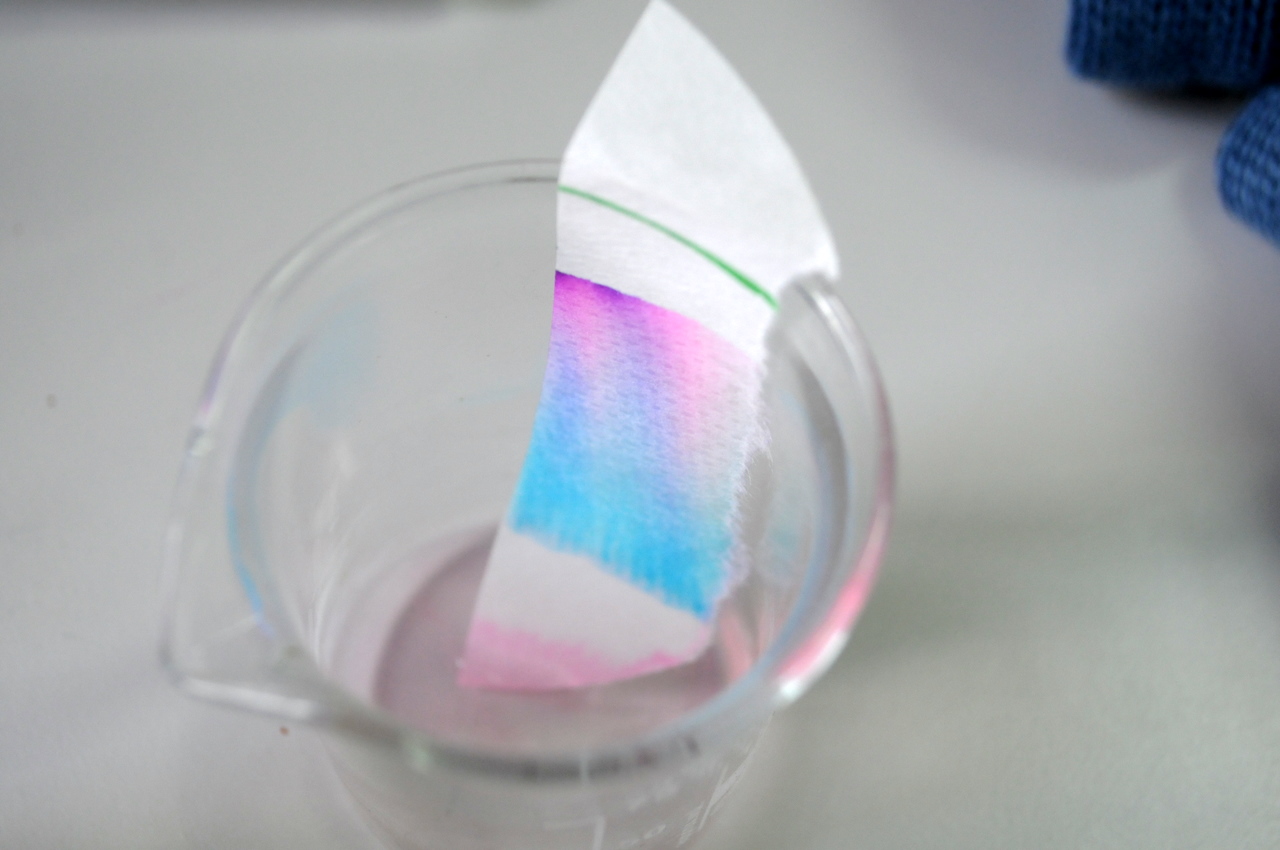This image is a rectangular photograph taken from above, looking down into a round scientific beaker. The beaker, which features a slightly pointed lip for pouring, contains a small amount of liquid at its bottom. A test strip is immersed in the liquid, with one end submerged. The strip is predominantly white with a gradient of colors: starting from the submersion point, it turns pink, then transitions to a rainbow block featuring pink, purple, and blue hues, and finally, a green stripe near the top. The beaker itself is placed on a white table, and in the top right corner of the image, a glimpse of a blue knitted material, likely part of someone's sweater, is visible.